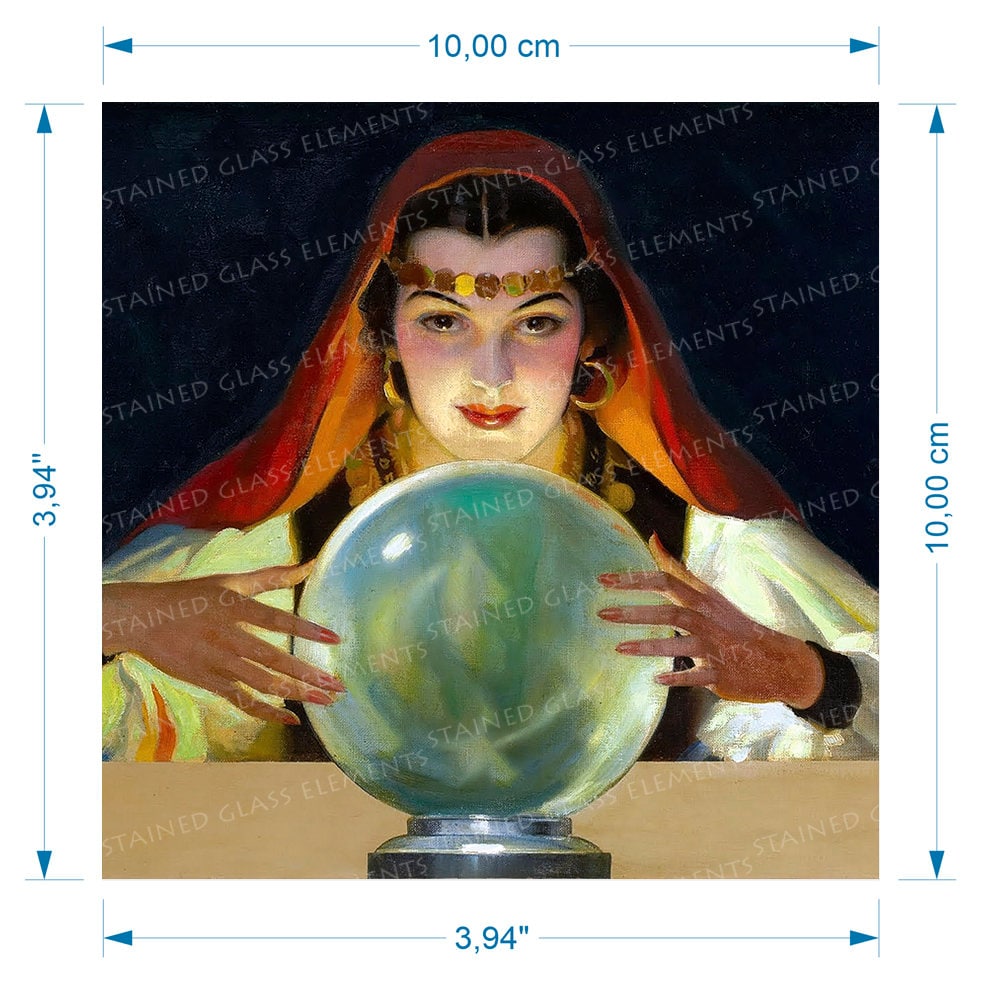This illustration portrays a classic fortune-teller, characterized by detailed elements and measurements surrounding the image. The woman at the center, assumed to be of Romani Gypsy heritage, gazes into a prominent crystal ball with both hands gently placed on either side. She dons a red shawl over her dark hair, a gold headband adorning her forehead, and large golden hoop earrings. Her expressive eyes and dark eyebrows add a touch of realism, while a gold chain peeks from around her neck. She wears a white blouse with voluminous sleeves under a brown cardigan or waistcoat. The image itself has a vintage style, further enriched with stained glass-like elements in hues of black, red, and greenish blues. The dimensions of the image are clearly indicated around the edges, marked as 10 cm by 10 cm and 3.94 inches by 3.94 inches, with arrows pointing to each side. These measurements stand out against a white background, which also features a slight diagonal watermark.